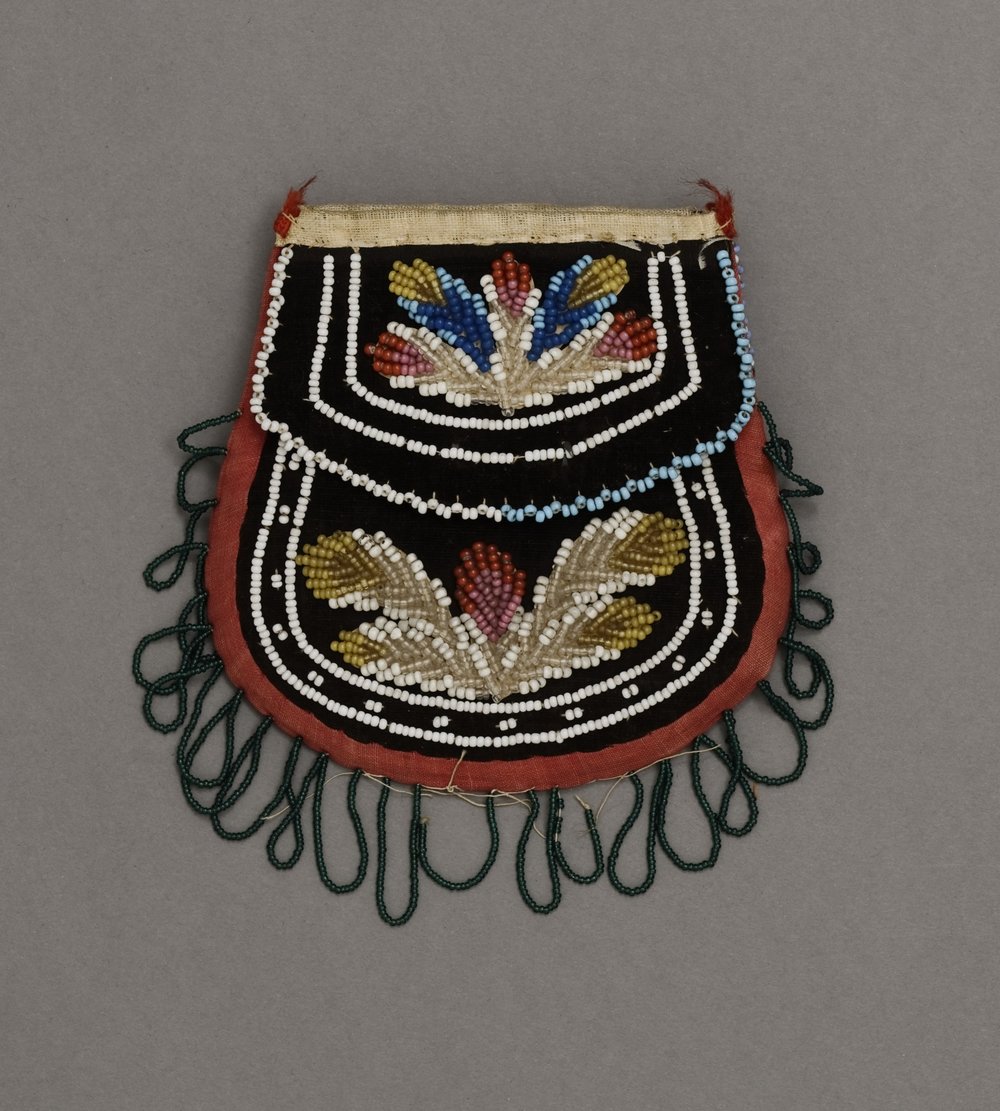This image showcases a detailed piece of handcrafted Native American beadwork, set against a solid gray background. The artwork appears to be a small beaded purse or clutch with a rounded shape and a straight top line, featuring a folding flap closure. The intricate beadwork on the flap displays a vivid dark blue section with patterns that resemble feather designs. Below the flap, the purse transitions into a red section accented by a small blue patch. This area also showcases intricate beading in beige, white, and maroon, continuing the feather-like patterns. Adorning the edges of the purse are decorative black beaded tassels. The bottom of the purse is embellished with a series of hanging fringe loops, possibly made of yarn, in a dark green hue. These elements come together to form a vibrant, ornamental piece that reflects traditional Native American artistry.